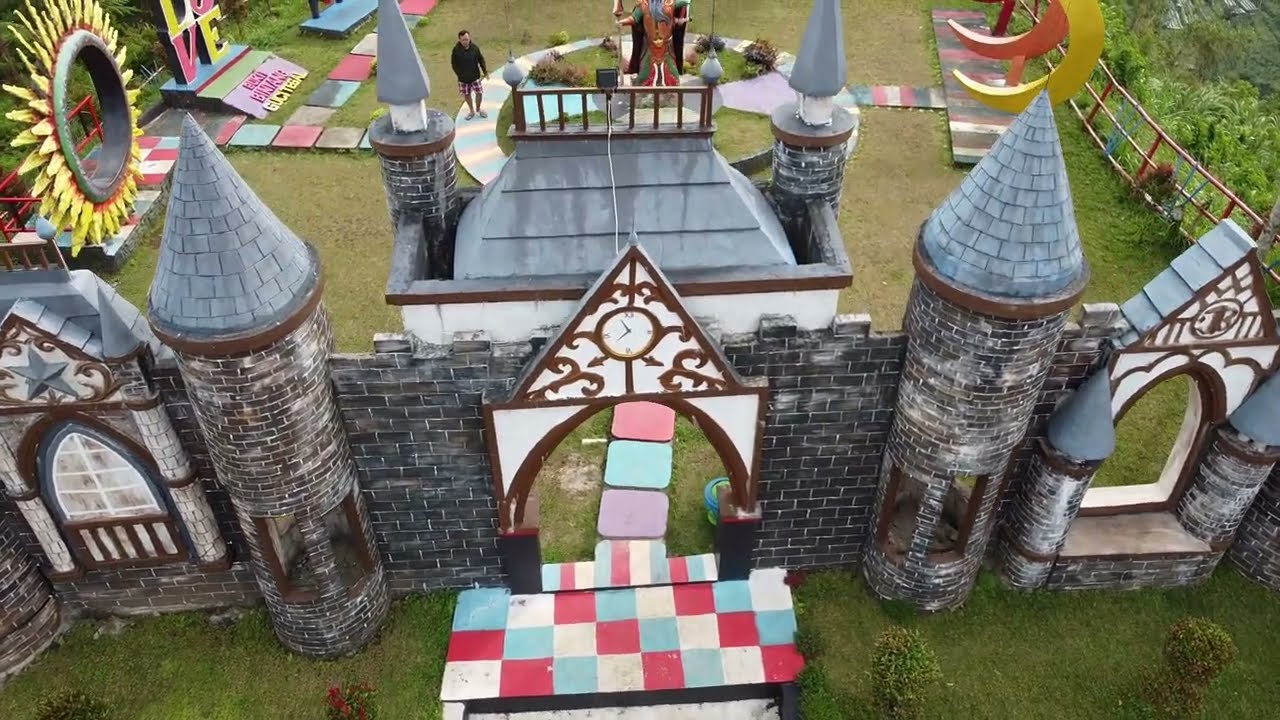The image depicts a whimsical, kid's style miniature golf course or a large-scale interactive board game with a distinct handmade artistic aesthetic. The forefront of the image features a colorful, flat, castle wall stretching horizontally at the bottom, with two columns topped with cone-shaped roofs flanking an arch-shaped door and a checkered floor leading into the castle's main entrance. Off to the top left corner, there is a large sunflower prop with yellow petals but no center, adding to the playful atmosphere. Behind the sunflower, the letters 'LOVE' are displayed in bold, large characters, with the 'L' and 'O' positioned above the 'V' and 'E.' The right side showcases wooden moon shapes, contributing to the artistic decor. The scene is set outdoors on grass, and a single person can be seen standing in the background, highlighting the scale of the setup. The pathway within the scene is vibrant, featuring various colors like white, blue, and touches of red, integrating seamlessly with the outdoor environment. The entire depiction suggests an imaginative space for people to walk around, explore, and enjoy, reminiscent of a playful amusement park or an elaborate theatrical set.